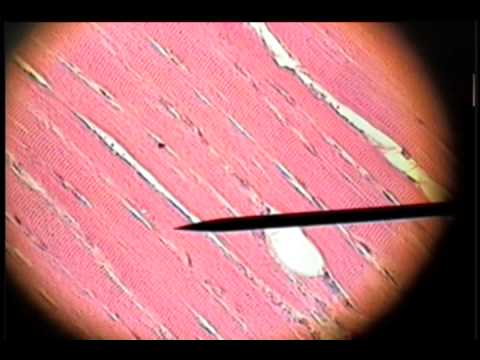This image, viewed under a microscope, presents a highly magnified circular area with a black background and a shaded black border around the edges of the circle. At the center lies a pinkish-red expanse, characterized by a series of white, striated lines that traverse through the red field, potentially indicating muscle tissue. Prominently featured is a long, sharp pointed object resembling the needle or pointer of the microscope, positioned towards the bottom half of the image, casting a faint shadow. The red area is marked by small beige stripes, with two significantly larger than the others, and a solitary cream-colored blob standing apart from the striations. Additionally, a small black speck is present, its purpose unidentified. The scene suggests a scientific or medical examination, possibly focusing on the structure or diagnosis of tissue.